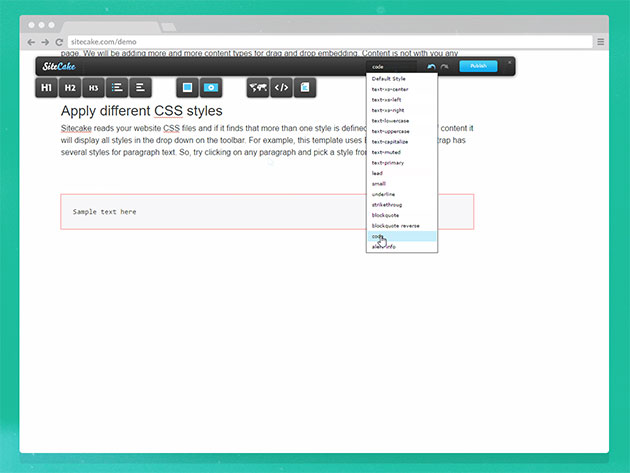The image depicts a web page with a thick green border surrounding it. The top section of the page is gray, housing three white circles. A white rectangular box intended for the browser URL appears blurry, but it faintly displays "somethingcake.com/demo." Below this, another text reads, "We will be adding more and more content," followed by some illegible text possibly related to drag-and-drop embedding.

A prominent black rectangle spans the width of the page, containing the word "SITE" in white text on the left end and "CAKE" in blue text on the right. Adjacent to this is a black search box where something has been typed, displayed in white. The search box appears to act like a drop-down menu with white contents and black text, but its specifics are unclear. A mouse cursor points to one of the options, which is highlighted in blue, but the text remains unreadable.

Further to the right, there is a blue rectangular button with an initial "P," likely indicating it says "Publish." Below this button, black text outlines functionality to "apply different CSS styles," mentioning terms like "site, cakes, read, share, website, CSS files" and explaining how multiple styles are presented in a drop-down if detected. It encourages users to click any paragraph to pick a style, which would open a pop-up block showcasing several paragraph styles.